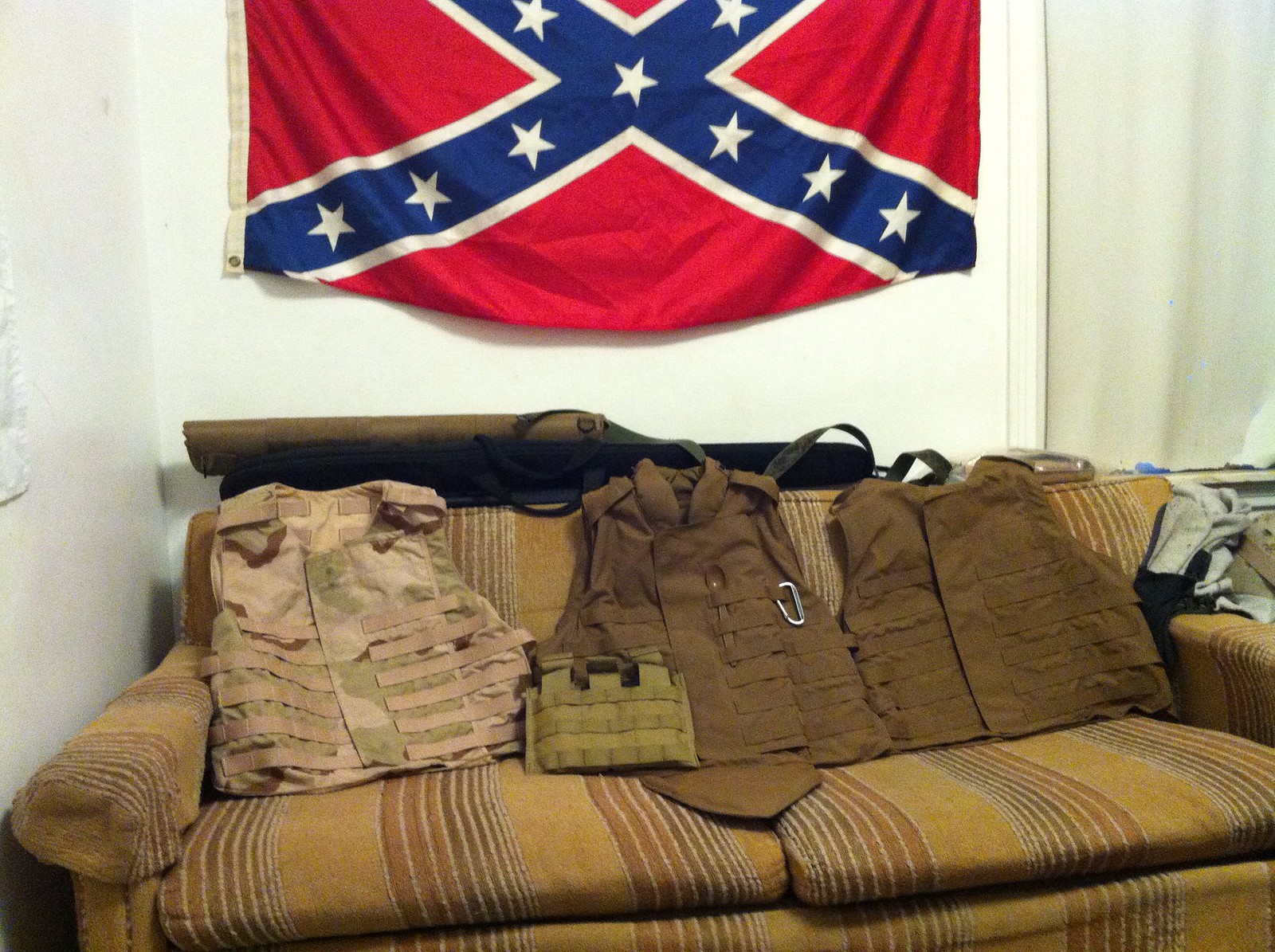This photograph captures a corner of a living room, showcasing a somewhat old and worn two-seater couch. The couch fabric, colored in a faded olive green with brown, red, and blue stripes, supports an array of tactical gear. Resting against its back are four bulletproof vests: one is desert camouflage with pale beige and sage green shades, another is solid olive drab green, and the final two are a darker brown or olive green. Additionally, a folded vest is positioned in front of the others, noticeable among the gear. Two soft rifle cases, one brown and one black, are tucked between the couch and the wall. The room's off-white walls feature a window draped with a white curtain, and prominently above the couch, a Confederate flag hangs. The flag is bright red with a navy blue X adorned with white stars crossing from corner to corner.